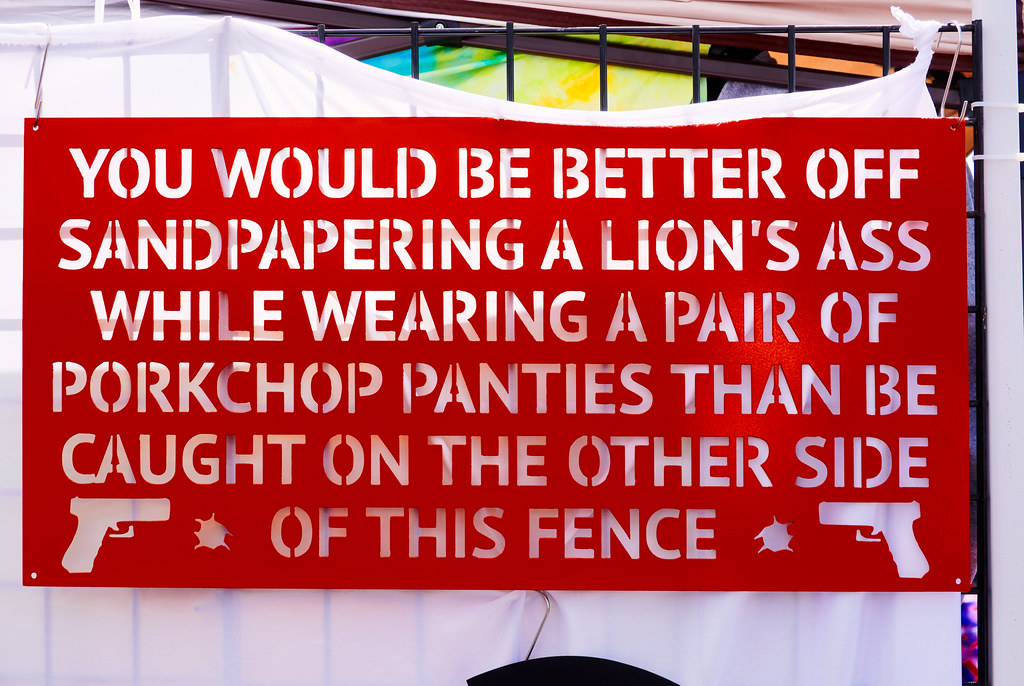The image is a color photograph in landscape orientation, showcasing a vividly detailed scene. In the foreground, there's a prominent red sign with intricate white lettering, mounted against a white sheet draped over a sturdy black metal fence. The sign reads, "You would be better off sandpapering a lion's ass while wearing a pair of pork chop panties than be caught on the other side of this fence." The text is rendered in a stencil-type font and spans six lines, emphasizing the warning message. At the bottom corners of the sign, there are white outline illustrations of pistols, with the gun on the left pointing right and the gun on the right pointing left. Adjacent to these pistols are small marks resembling bullet holes. The sign's stylistic choice of representational realism adds to the gravity and visual impact of the warning.